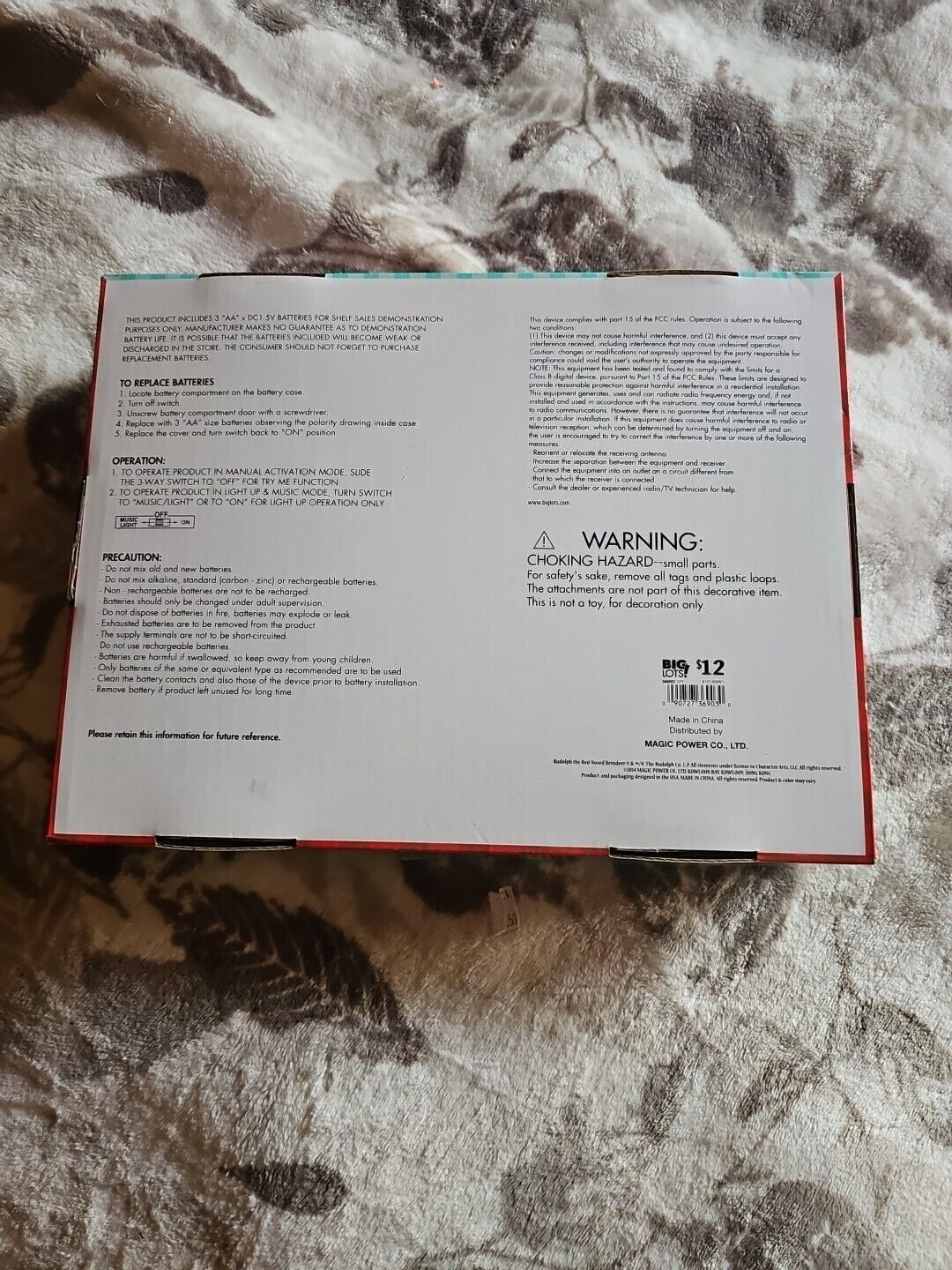The image is a close-up of the back of a product box, placed on a bedspread with a gray background and brown leaf patterns. The box prominently features a bold warning label indicating a choking hazard, suggesting that the product contains small parts unsuitable for young children. Below this warning, the print denotes the product was purchased from Big Lots for $12, featuring Big Lots' logo and a barcode. The text also includes instructions for replacing the three AA DC 1.5 batteries, cautioning that demonstration batteries in the store may be weak and advising customers to purchase replacements. Detailed steps for replacing the batteries and operating the product are listed, including safety precautions. Additional notes clarify that the item is decorative and not a toy, emphasizing the importance of removing all tags and plastic loops for safety reasons. The box is turned upwards, facing the camera, making it difficult to identify the exact product. The manufacturer's information also mentions it is distributed by Norla Magic Co. and made in China. The setup is against a white and gray embroidered cloth with leaf designs, contributing to the monochromatic theme of the photograph.